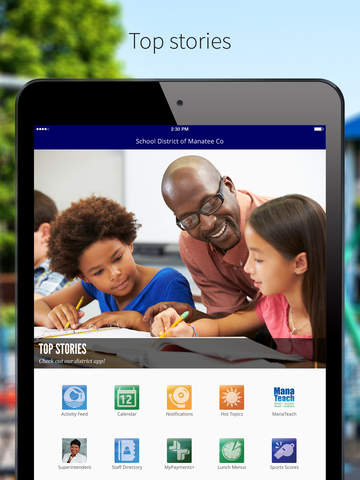A potential image caption could be:

"A digitally created image, possibly a screenshot, features the interface of a web page or an application displayed on a smartphone. The backdrop showcases a serene blue sky and leafy green trees in the distance, providing a pleasant, yet indistinct, background. The focal point is the smartphone screen, which has a black border at the top displaying the title 'Top Stories.' Prominently displayed is an image of a smiling Black man wearing glasses. He is engaged in a teaching moment, looking down at a student with long dark hair and honey-colored skin, who is holding a pencil and pointing at a notebook on a desk. Beside her, another student, a Black girl with short curly hair, also holds a pencil and attentively focuses on the notebook. Below the image, the section is labeled 'Top Stories' with additional text that is too small to read clearly. The bottom of the screen features several tiny icons symbolizing different functions, such as a calendar, weather updates, a doctor in a white coat, and a clock. Despite the small text, the graphical elements suggest a variety of options available to the user."